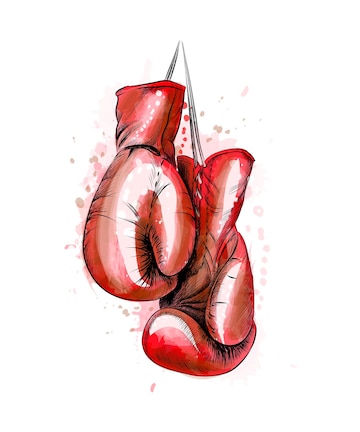This image features a water painting of a pair of red boxing gloves hanging in the center. The gloves, marked by white reflections that create a horseshoe shape on the thumb and the thicker part of the hand, are detailed and vivid. They hang from white strings that appear to be part of the gloves themselves. The glove on the left side of the image is the right glove, showing a few black markings, while the glove on the right side of the image is the left glove, with the palm facing forward and appearing slightly brownish in the palm area. The all-white background is interspersed with delicate specks of watered-down red paint that have a pinkish hue, adding depth and texture to the scene. There are no texts within the image, keeping the focus solely on the hanging gloves.